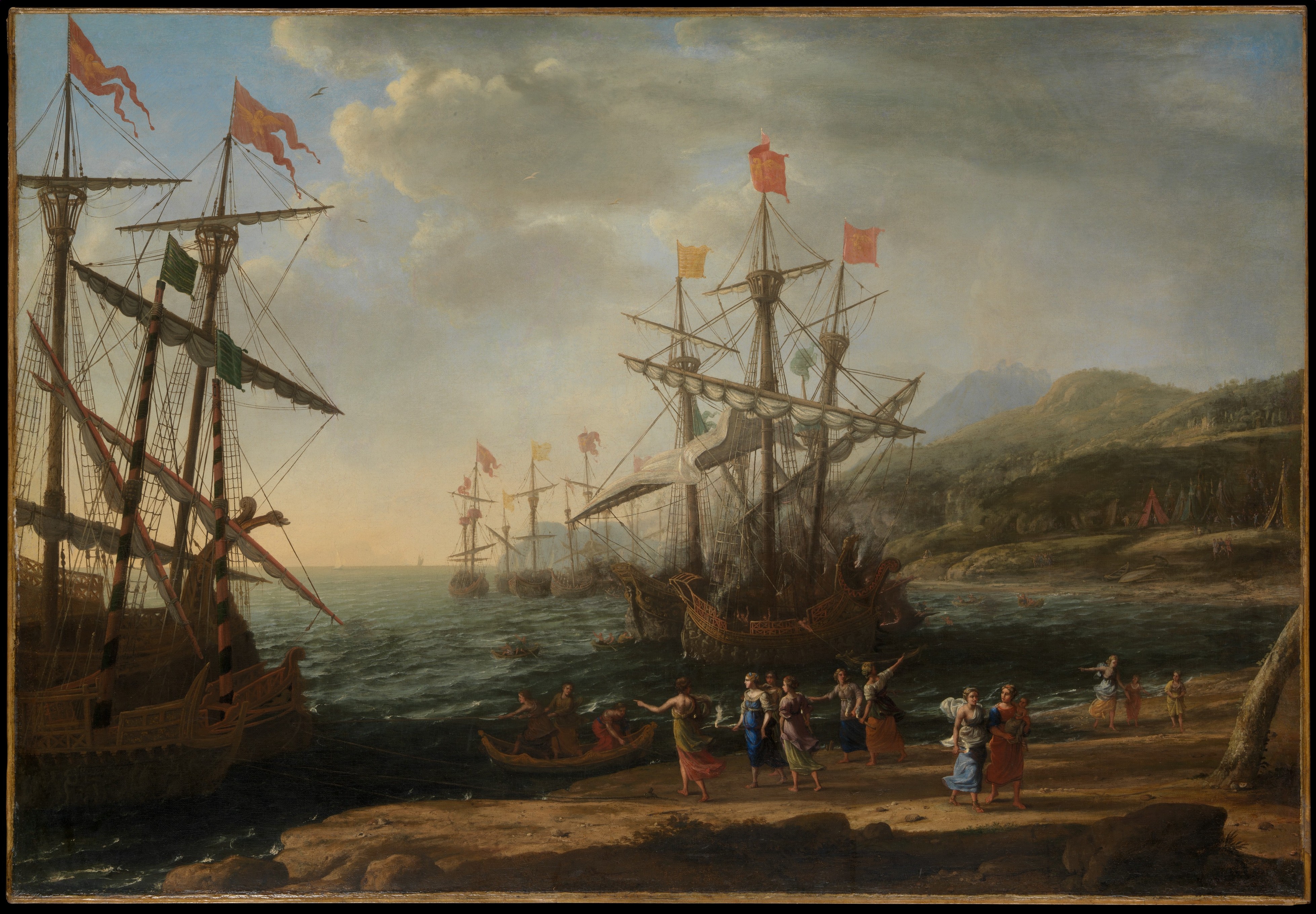This evocative oil painting, likely from the late 18th or 19th century, captures an atmospheric coastal scene reminiscent of J.M.W. Turner's dramatic style. The foreground features a rocky beach with a dozen or so women and children, dressed in long summer dresses, waiting barefoot for their loved ones to return from sea. Amidst a backdrop of turbulent, fog-laden waters and imposing hills, the composition is balanced by a fleet of multi-masted schooners and wooden ships coming into a cove. Some ships are closer to shore with rowboats making their way toward land, one boat having just landed. The scene is bustling with maritime activity, accentuated by dramatic clouds and choppy waves. On the left side of the beach, a collection of teepees hints at a diverse cultural presence, making the painting both lively and richly detailed. The overarching narrative is one of anticipation and reunion as seafarers approach the shore, embraced by the dramatic and natural grandeur of both sea and land.